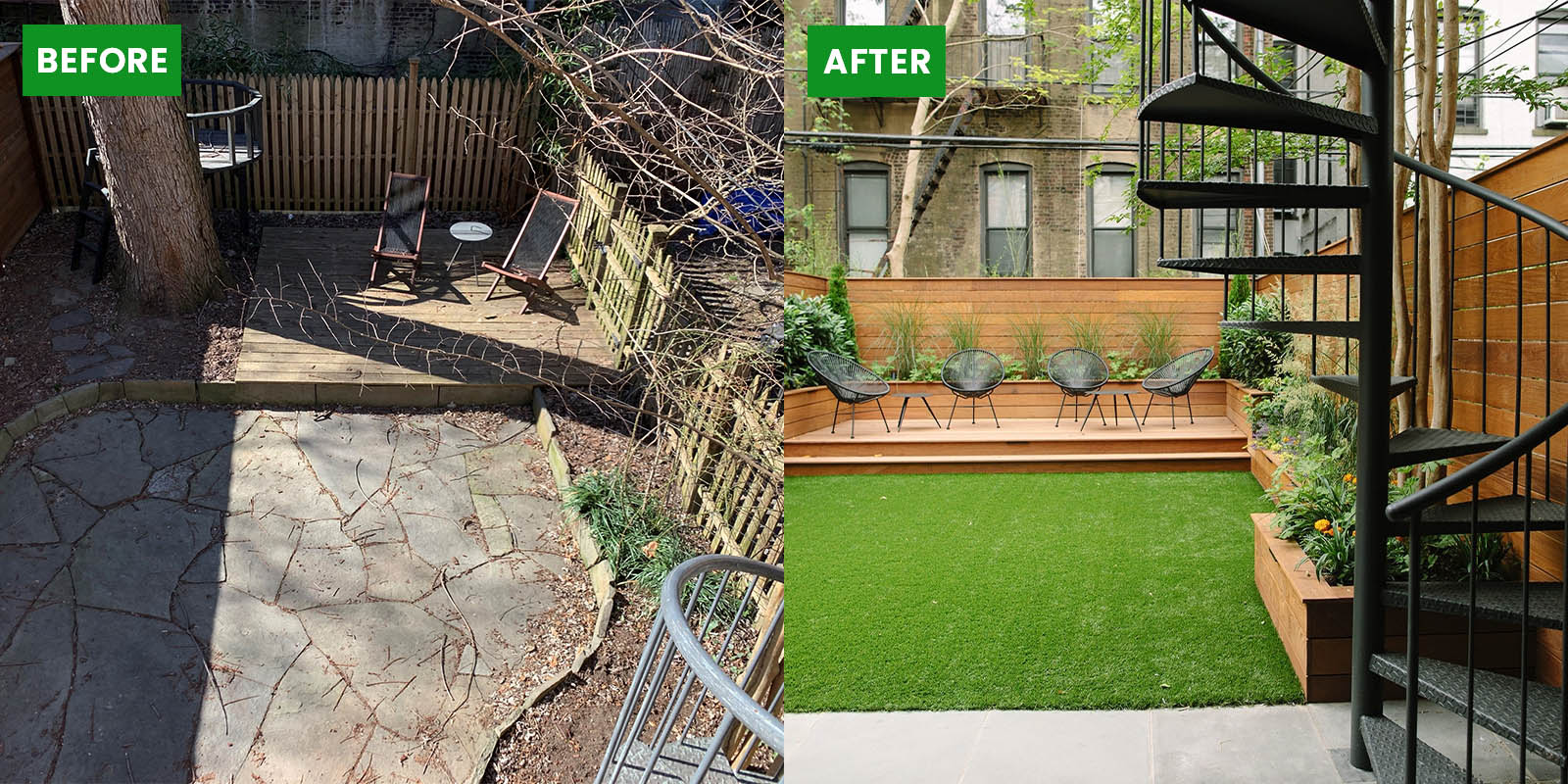In this two-pane photo set, we have a transformative before-and-after depiction of an urban backyard. The 'before' image, marked with a green label in the upper-left corner, showcases a gray, cracked concrete patio dominated by a large cement pillar and the trunk of a dead tree on the back left. A small wooden platform in the back right supports a rusted, lonely patio set of two chairs and a white table. The dilapidated picket fence on the right side seems ready to collapse, with a silver-gray spiral staircase peeking into the view. The overall look is desolate and uninviting.

The 'after' image, labeled similarly, captures a stunning transformation into a vibrant urban oasis. The once desolate concrete ground has been replaced with luscious, vivid-green artificial turf. The previous wooden platform has been updated to a medium brown deck, framed by a horizontal paneled wood fence that provides additional height and privacy. This new fence is orangey-tan and much more aesthetically pleasing.

The black spiral staircase, now refurbished and sophisticated, contrasts beautifully with the fresh surroundings. Potted plants in square wooden planters and a row of green and orange flowers create a lively ambiance. The raised wooden deck area, accessed by two steps, features four elegant, black metal chairs positioned around two tables, making it perfect for social gatherings. The backdrop of the scene shows the windows of a neighboring building, hinting at the urban setting while ensuring a sense of seclusion and peace. This comprehensive makeover has turned a rundown space into a beautifully appointed urban retreat.